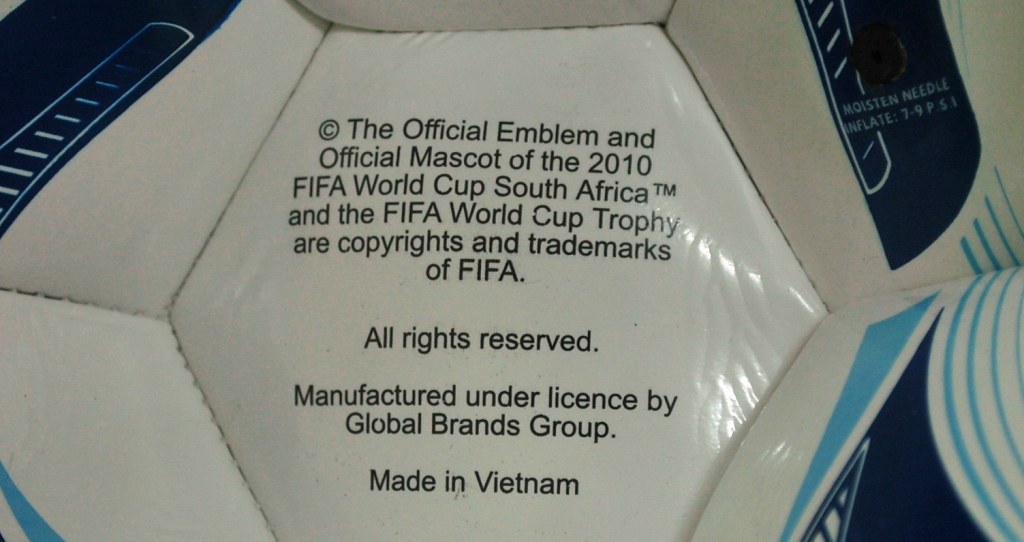This color photograph, oriented in landscape, features a unique sports ball prominently in the center. The ball's design incorporates a blend of white with blue detailing, creating a visually striking composition. The object, appearing to be a six-sided structure, reveals its contents slightly flared open, exposing a white central section adorned with black text. The inscription reads: "The official emblem and official mascot of the 2010 FIFA World Cup South Africa, and the FIFA World Cup trophy are copyrights and trademarks of FIFA. All rights reserved. Manufactured under license by Global Brands Group. Made in Vietnam." The text is neatly centered in separate paragraphs. Additionally, the ball includes instructions for inflation, specifying "moisten needle, inflate 7-9 PSI." The photograph captures the intricate seam work and the inflating needle insertion point, reflecting a high level of photographic realism. The overall aesthetic of the image is representative realist, emphasizing the detailed craftsmanship of the ball.